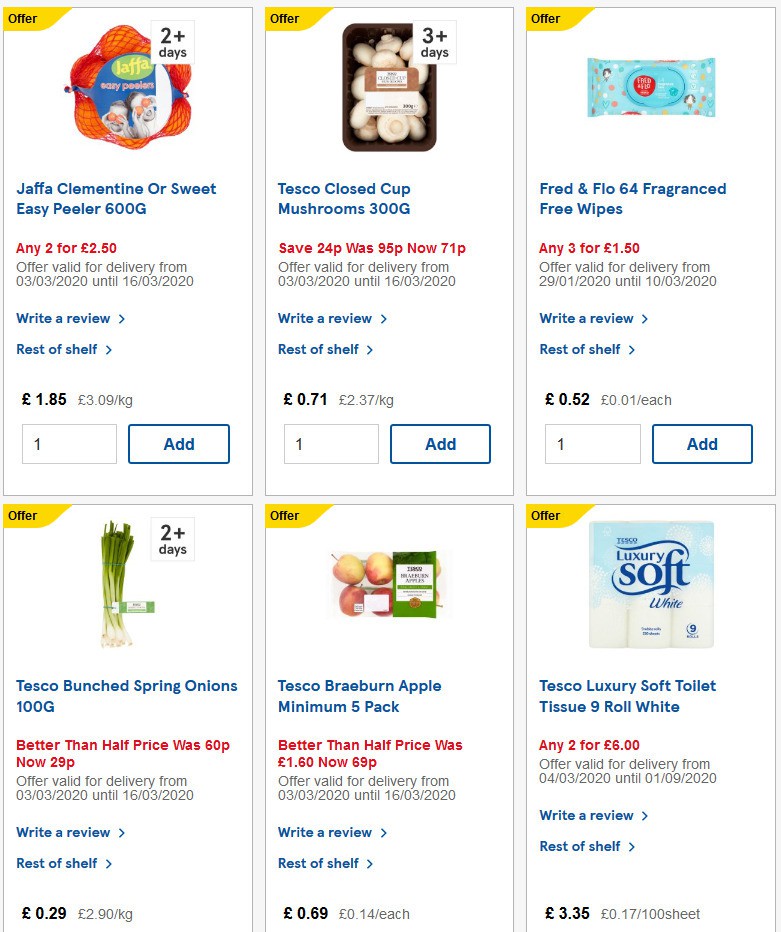The image features a white background with six product boxes, each displaying a distinct product along with a detailed description and price. On the top left corner of each product box, there is a yellow tag that reads "Offer." The first product, located in the top left box, shows a bag of oranges labeled as "Jaffa Clementine or Sweet Easy Peeler, 600 grams." The special offer for this product is "Any two for £2.50," valid for delivery from 03/03/2020 until 16/03/2020. Below this, users can find hyperlinked text options to "Write a review" or view the "Rest of shelf." The price under this specific product is £1.85, equating to £3 per kilogram, with an adjacent button outlined in blue that says "Add."

To the right of this product, another box highlights "Tesco Closed Cup Mushrooms, 300 grams," showing a price reduction—originally costing 95 pence, now available for 71 pence, resulting in a savings of 24 pence.